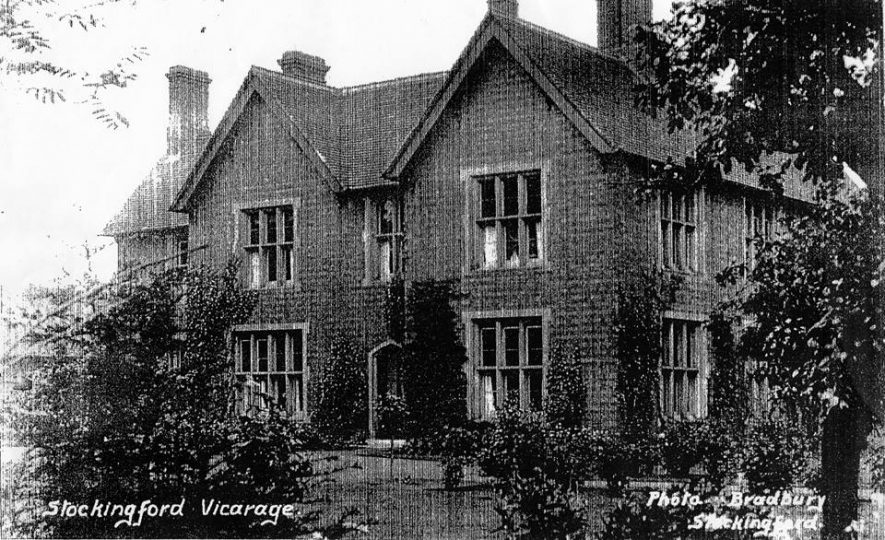The black-and-white photograph captures an expansive and symmetrical mansion, identified by the text in the bottom left as "Stockingford Vicarage" and attributed in the bottom right to "Photo Bradbury Stockingford," indicating its historical nature. The mansion, likely over a century old, features a robust, well-constructed design with numerous tall windows distributed evenly across its two stories—eight on the bottom left, six on the bottom right, and six each on the upper left and right, with an additional four central windows above a dark front door. It is constructed from what appears to be brick or block and is surrounded by manicured lawns, trees, shrubs, and ivy climbing its sides. Four prominent chimneys rise from the steep gabled roof, suggesting multiple fireplaces within. The clear sky and sunlight shining on the mansion add clarity to the historical charm of this grand estate.